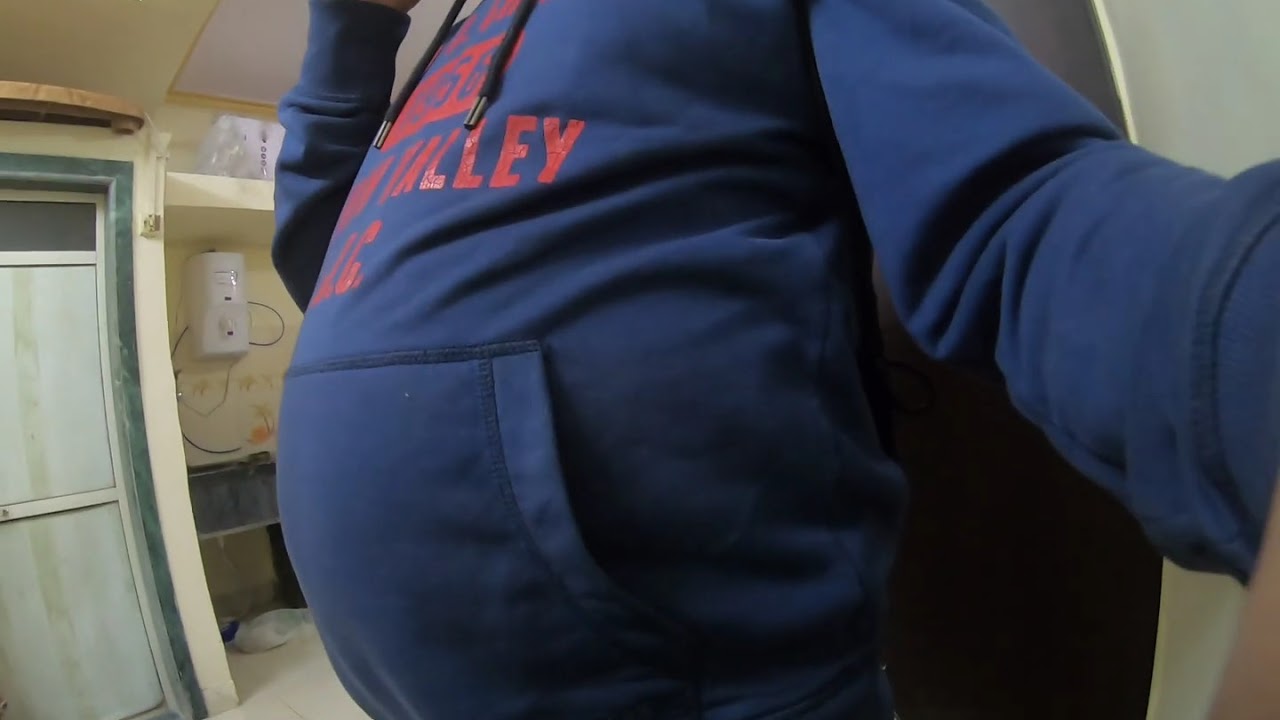A close-up photograph captures a person taking a selfie in what appears to be an old, poorly maintained bathroom. The image focuses on the torso, showing an overweight individual dressed in a large, dark blue hoodie with unreadable red text on the front, except for the word "valley." The shot is cropped oddly, excluding the person’s head and lower body, with one arm extended upwards, likely holding the camera. The background reveals faded yellow walls and a green door that's ajar, adding to the rundown appearance. A soap dispenser or drying machine is visible on the wall in the distance.